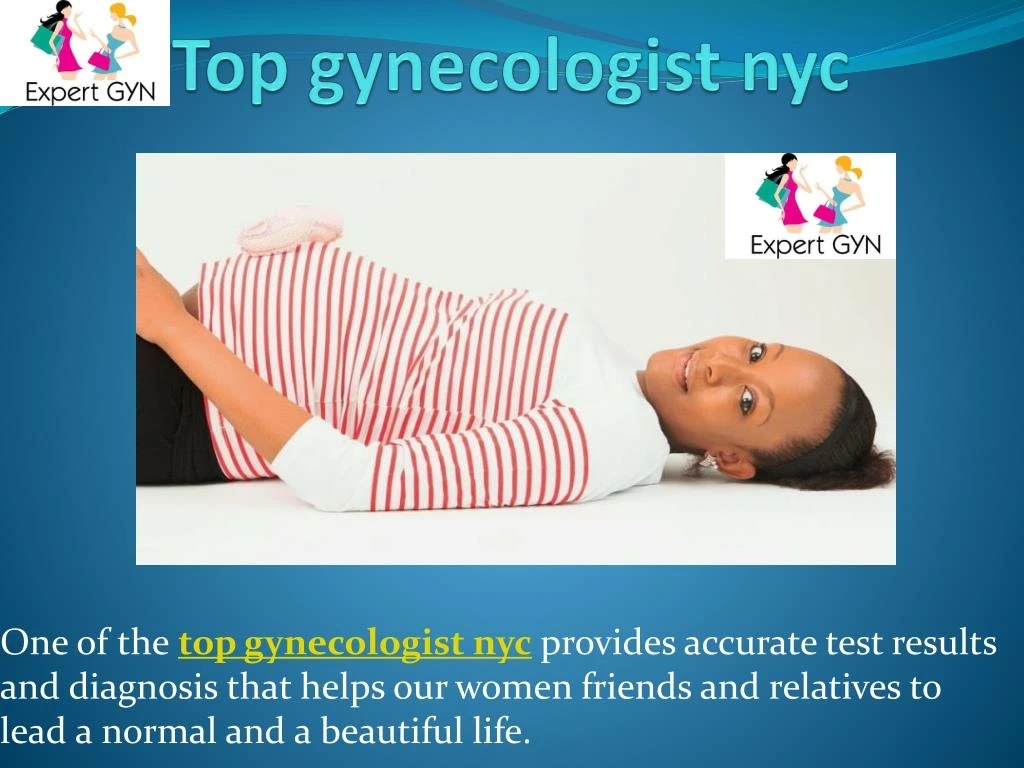This PowerPoint slide, designed with a gradient background transitioning from dark blue to light blue, features a detailed presentation on gynecological expertise. At the top left corner, there are illustrations of two cartoon women: one with long black hair wearing a purple-violet dress, and the other with long blonde hair in a ponytail wearing a blue dress, accompanied by the text "Expert GYN." Centered at the top in light blue font is the title "Top Gynecologist NYC," overlaying subtle digital wave patterns. Dominating the middle of the slide is a large photograph of a dark brown-skinned woman with black hair, possibly in her 30s or 40s, lying on her back and smiling at the camera. She appears to be pregnant, dressed in a shirt featuring horizontal red stripes with a white collar and white sleeve details at the elbows, set against a white backdrop. Below the image, in white text with "Top Gynecologist NYC" highlighted in yellow and underlined, the caption reads: "One of the Top Gynecologists NYC provides accurate test results and diagnosis that helps our women, friends, and relatives to lead a normal and beautiful life."